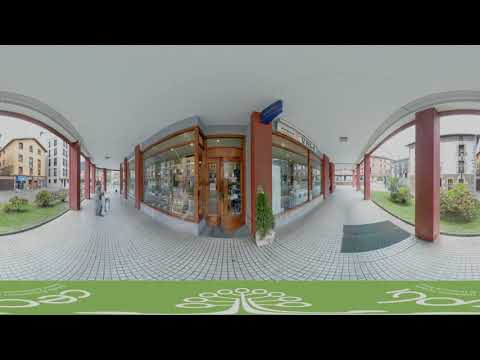In this fisheye lens image of an outdoor shopping mall, a variety of objects and vibrant colors are captured, creating a detailed and lively scene. At the bottom of the image, a green border runs across, adorned with white tree logos, set against a black line that extends across the top and bottom of the frame. This seems to highlight the setting's emphasis on nature and design. 

The central focus of the image is a walkway paved with white tiles, giving an impression of curving due to the lens effect. The walkway is flanked by a building with a red and white trim exterior, featuring a wooden door at its center and large glass windows that display items for sale inside. In front of this door, a small green tree sprouts from a white base, contributing to the greenery scattered throughout the scene, including various bushes and trees.

To the right, there is another red post supporting a white ceiling, while the ground showcases a black mat among the tiles. Additional storefronts, predominantly in colors of yellow and tan, extend across the mall area, evoking a welcoming atmosphere. On the left side of the image, residential buildings are visible, distinguishable by their numerous windows and possibly brick walls.

In the outdoor setting, under broad daylight, people are engaged in window shopping, with notable details like a man dressed in gray walking a white dog on the sidewalk. This vibrant scene captures various elements displayed in a collective and immersive outdoor shopping center.